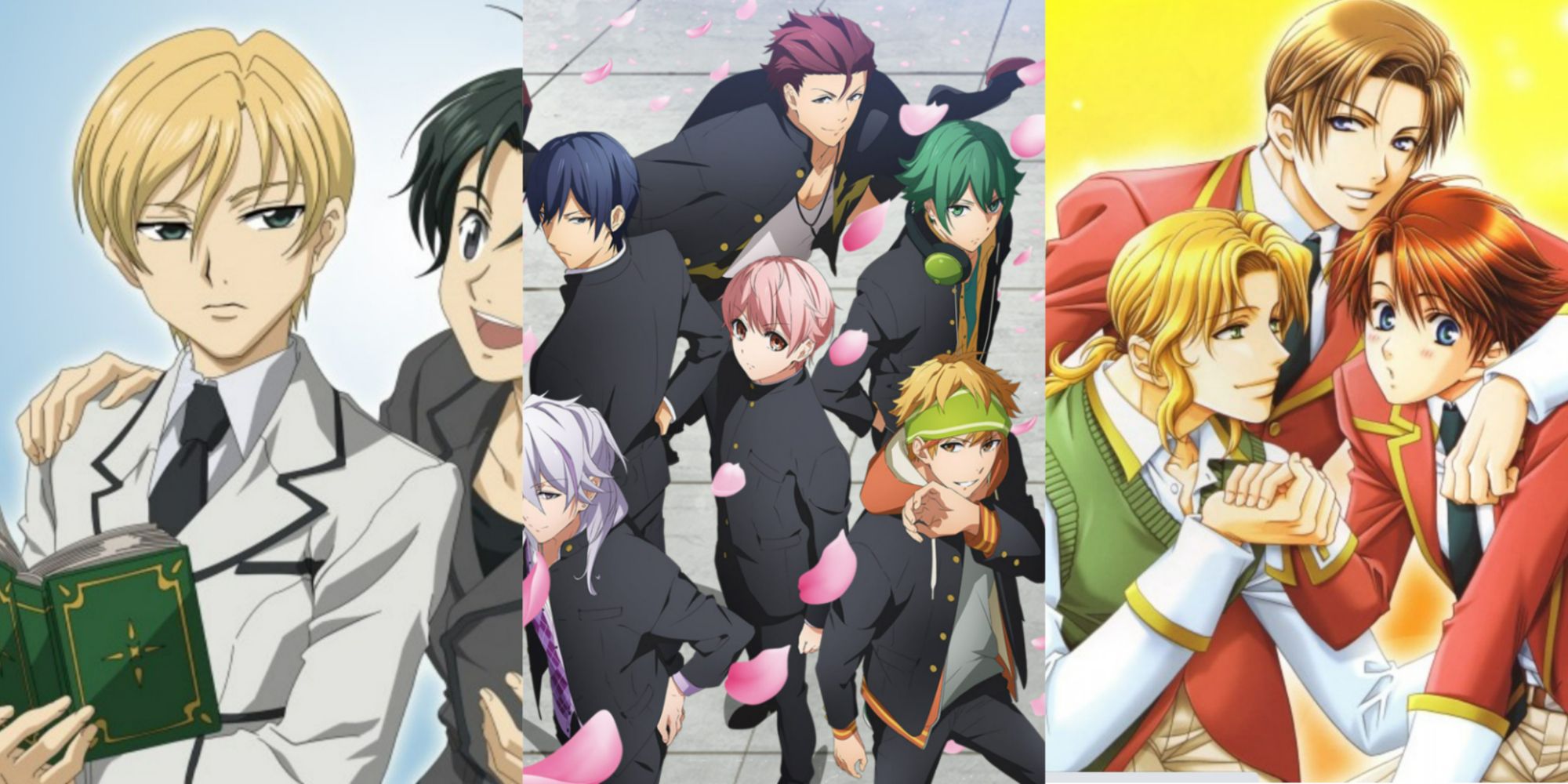This image showcases a triptych of anime illustrations, each panel enriched with distinct details. The left panel features two young men; the one in the foreground has blonde hair and is wearing a gray suit jacket with blue trim, a gray collared shirt, and a black tie, holding a green book. Standing behind him is another man with black hair, dressed in a gray jacket, his hand resting on the first man's right shoulder, seemingly engaged in conversation. The middle panel depicts a group of six characters, all adorned in gray or black jackets, highlighted by a variety of vibrant hair colors including purple, green, and pink. The central figure with purple hair is surrounded by five others, each with unique features like buttons on their jackets or additional garments like hoodies. The right panel presents three characters set against a yellow background: a blonde girl in a green cardigan holding hands with a boy wearing an orange jacket with gold borders, who is looking slightly toward the viewer. Behind them, another male figure, in a matching orange jacket and with brown hair, embraces the boy from behind, resting his hand on his shoulder. The absence of text allows the expressive attire, postures, and interactions of the characters to convey the narrative within this vividly detailed anime artwork.